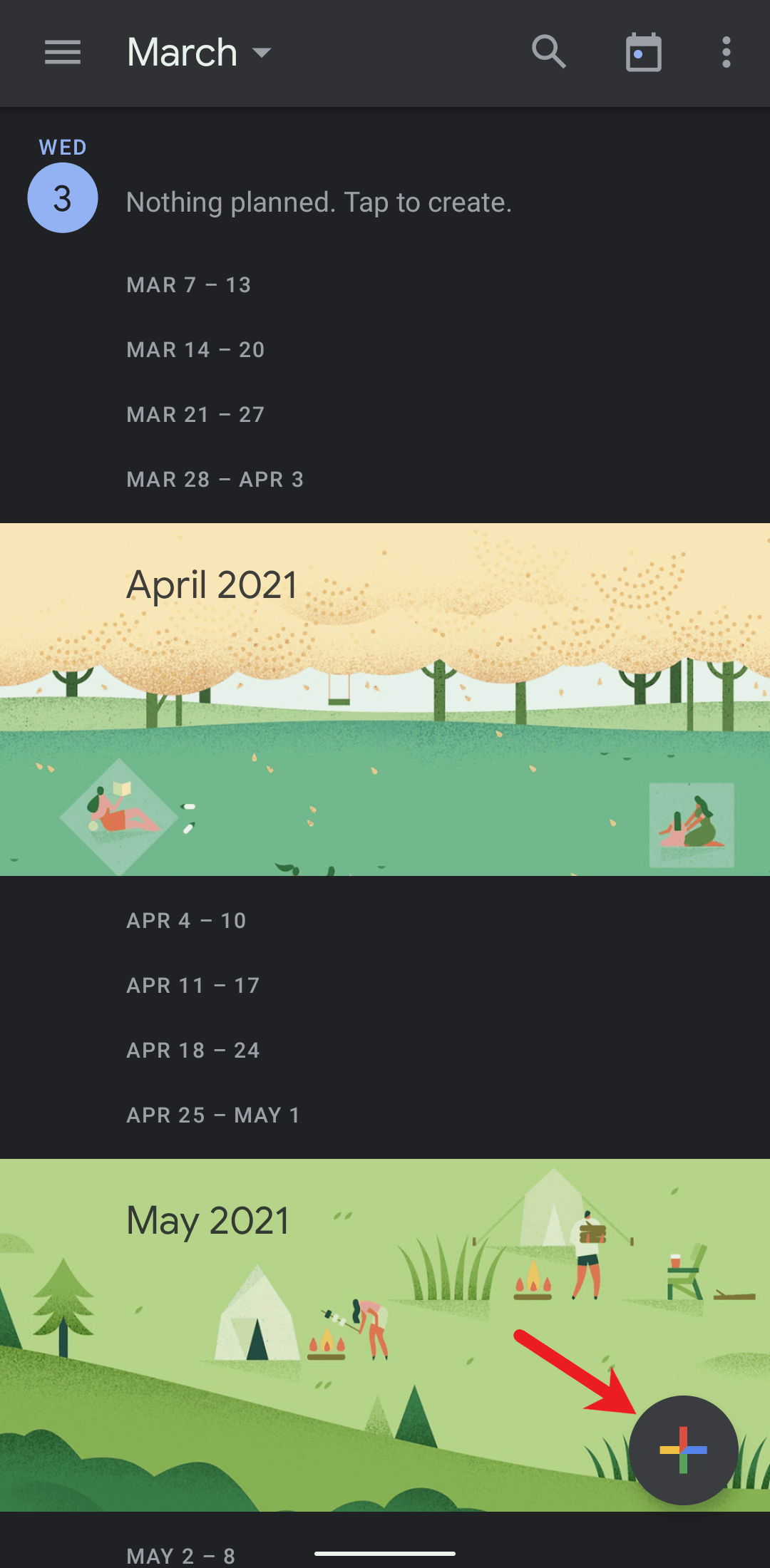Here is a cleaned-up and detailed caption for the image:

---

This screenshot from a mobile phone displays a calendar app interface. At the top is a gray navigation bar. In the upper left corner of this bar are three horizontal gray lines organized vertically, which likely represent a menu icon. Immediately to the right of the menu icon, the month “March” is displayed in white font, accompanied by a small gray arrow pointing downward, suggesting a dropdown menu. Further to the right are icons for a magnifying glass (search function), a calendar, and three vertical gray dots (options menu).

Below the navigation bar, in the upper left corner of the screen, a black rectangle contains the text “Wednesday” in blue uppercase font, abbreviated as “WED.” Directly beneath this text is a blue circle with the number “3” in black font, denoting the date. Adjacent to this circle, in white font, the text reads “Nothing Planned, Tap to Create,” providing users with an option to add new events.

The following section is divided into weekly segments listed by date ranges: “March 7-13,” “March 14-20,” “March 21-27,” and “March 28-April 3.” Below these date ranges is a colorful graphic depicting trees and people relaxing on mats in a park, serving as an illustration for the month of April 2021. Following this image, the calendar displays additional weekly date ranges within black rectangles: “April 4-10,” “April 11-17,” “April 18-24,” and “April 25-May 1.”

Next, the month “May 2021” is labeled, followed by the specific date of “May 28.” Below this, another graphic showcases people camping on grass, providing a thematic backdrop for the date.

---